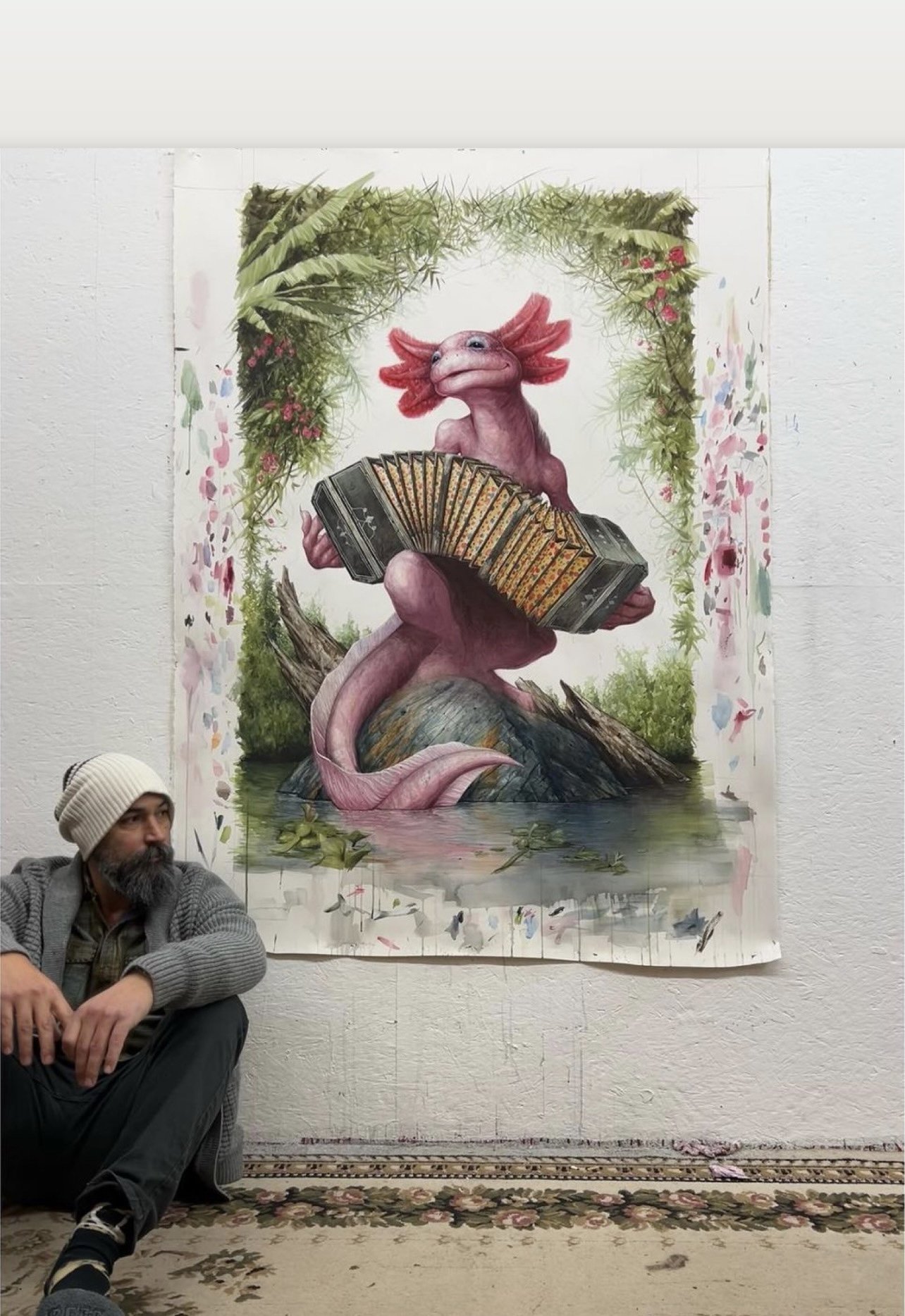This color photograph captures a detailed image of a painting on a white concrete wall, enhanced with delicate striations. The painting, prominently featured within a white bordered poster, depicts a serene natural scene: A pink axolotl, characterized by its distinctive flared gills and human-like limbs, sits on a boulder by a creek. The axolotl is playing an accordion, complete with human-like pink fingers, and is surrounded by reflective water that flows around green plants and a wooden log protruding from the creek. The background of the painting is predominantly white, showcasing tufts of greenery on both top corners and additional foliage emerging around the boulder and decaying log structure.

In the bottom left corner of the photograph, a man, possibly the artist, is seated on a tan floor rug against the white wall. He is dressed in a gray sweater, a beige knit hat pulled over his ears, and black pants, complemented by black sneakers. His hands rest upon his bent knees, and he looks contemplatively towards the right. The detailed juxtaposition of the painting and the man evokes an intimate gallery atmosphere, emphasizing both the intricacies of the artwork and the reflective mood of the observer.